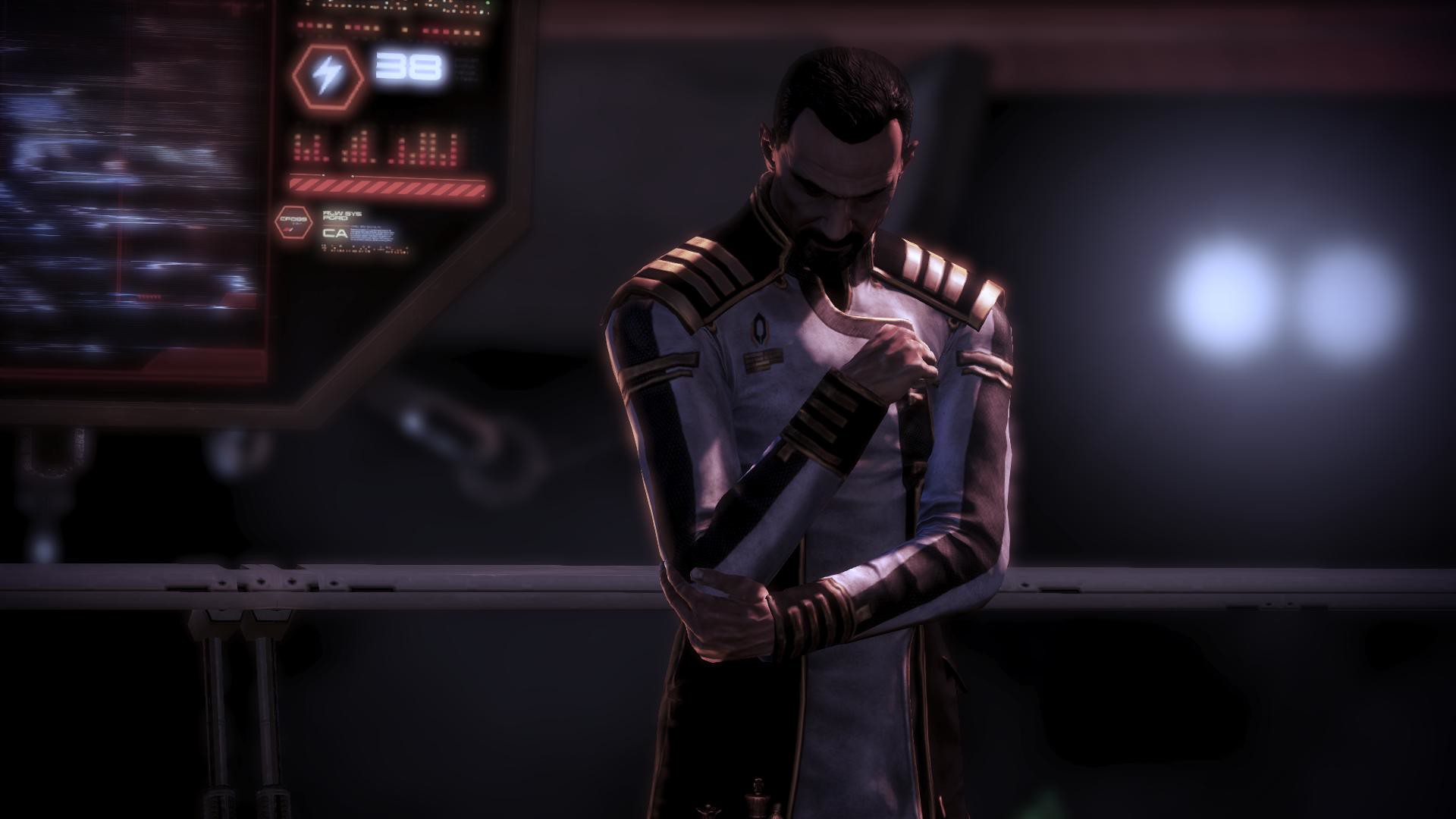The image appears to be a 3D rendering from a video game, featuring a man dressed in a military-type officer uniform. He stands in the front and center, holding his right arm slightly over his heart with his left hand gripping his elbow, as he looks down pensively. He has short black hair, dark eyebrows, and a neatly-kept black beard. His attire is a long coat that is silver and dark brown, adorned with gold bands that cross his shoulders, reminiscent of representative epaulets. The background is dimly lit, suggesting a setting that might be a spaceship or high-tech facility. Behind him, there is a railing and machinery with various lights and symbols. Notably, on the left side, there is a digital screen displaying a lightning bolt sign, an octagonal shape, a red glaring number 38, and some graphs. Additionally, on the right side of the image, there are blurred headlights, adding to the high-tech ambiance.